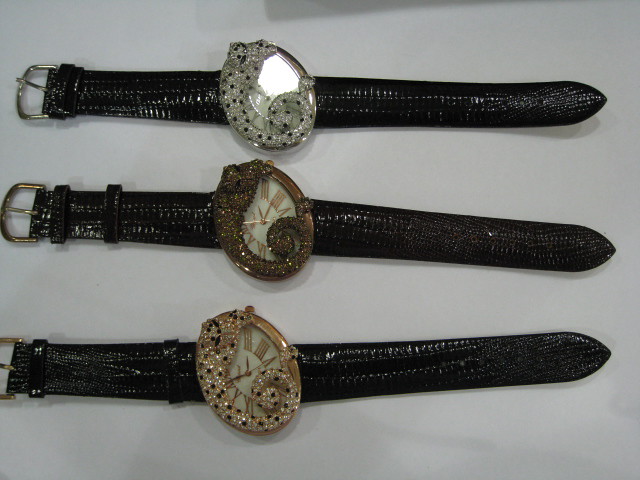The photograph displays three intricately designed wristwatches, each adorned with elaborate lizard motifs and set against a white background. All three watches feature dark leather alligator skin straps that are fastened with buckles—two gold and one silver—positioned to the left. The watch faces are oval-shaped and encrusted with crystal gems, making it challenging to tell the time. The top watch, with a black band, showcases a silver lizard with black dots, its body and tail coiling around the glass face. The middle watch, also with a black band, features a brown lizard in a similar coiled pose. The bottom watch has a golden lizard with black dots, also coiling around the golden watch face, adding a decorative touch. Despite being functional timepieces, each watch serves more as an ornate accessory due to the elaborate lizard designs that obscure the watch faces.